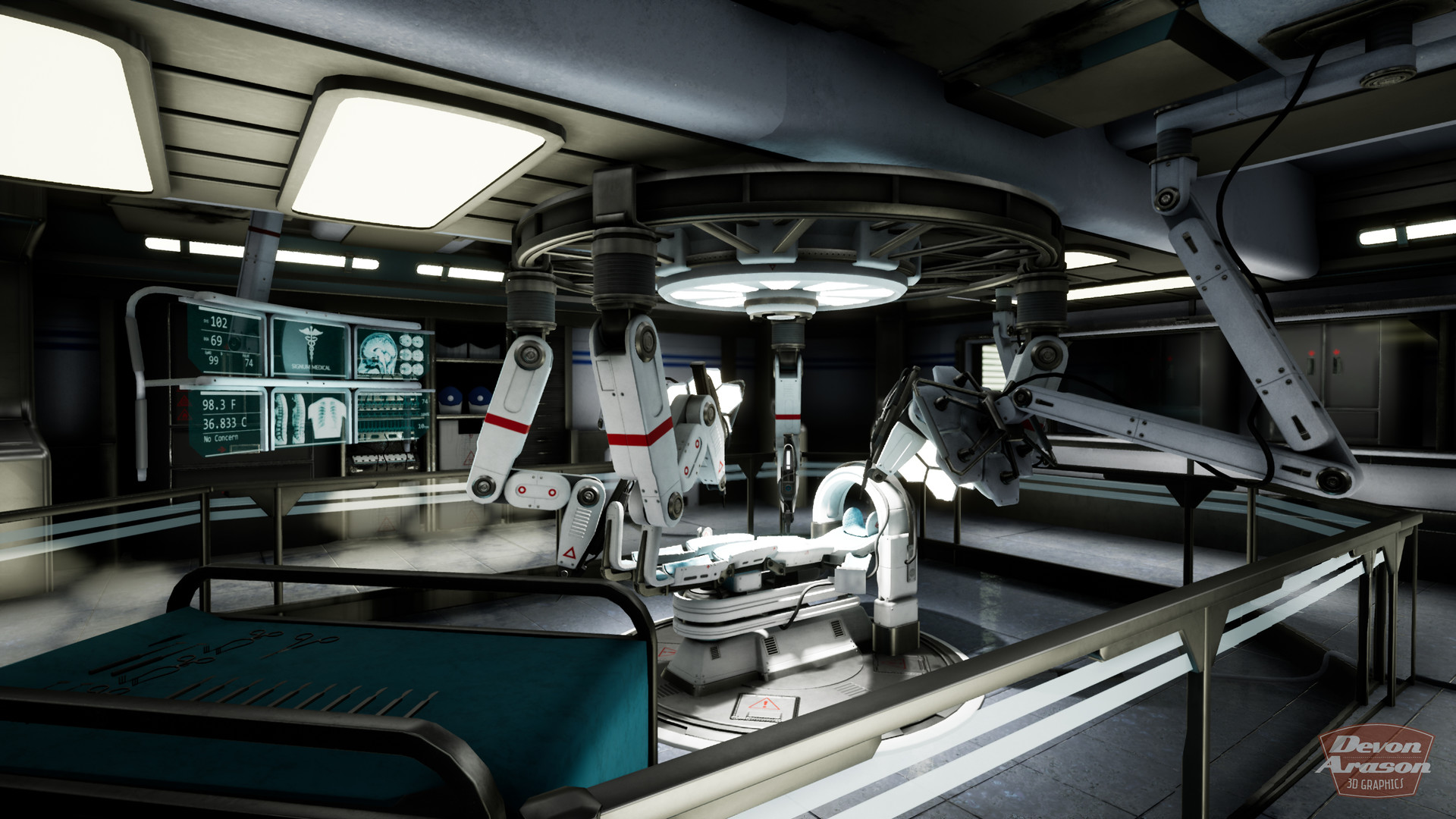The image depicts a highly advanced, technologically sophisticated medical room, likely within a futuristic or space-bound setting. Central to the scene is a large, metallic operating table with a semicircle device over the top, designed for a patient to lie beneath. Surrounding the table are numerous robotic arms poised for surgery or medical intervention. The ceiling features built-in lighting and a circular device that seems to beam light down onto the table. To the left, a screen displays medical diagnostics, including vital signs and x-rays. The room's aesthetic is predominantly silvery-gray with some blue-turquoise and red accents, reinforcing the clinical atmosphere. Notably, the room is bordered by metal railings, suggesting either a viewing gallery or a display setup, which, along with the inclusion of a cart with surgical tools, implies a cutting-edge medical laboratory. Adding to the artificial ambiance, the image carries the logo "Devin Arasin 3D Graphics," indicating a computer-generated design.